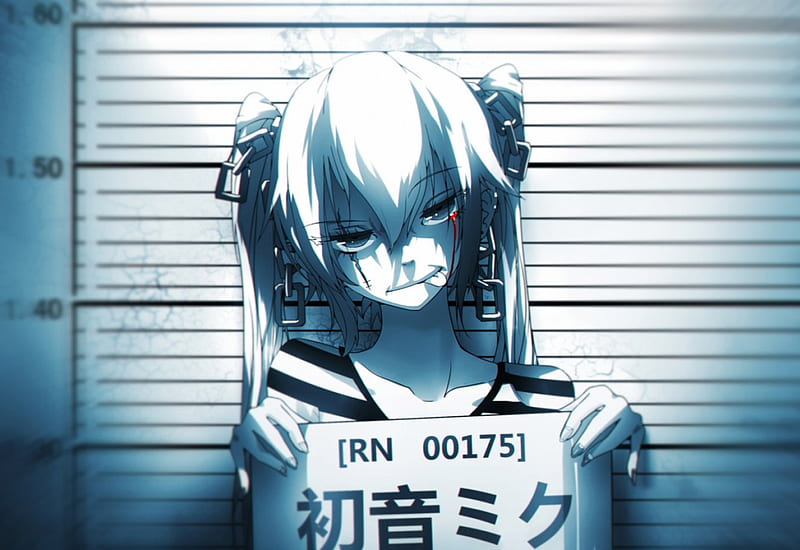This is a detailed digital image of a Japanese anime girl taking a mug shot. The girl has distinctive long, white hair styled in pigtails that are held up by large metal chains instead of hair ties, allowing them to hang. Her bangs fall down the front of her face, framing her large, half-lidded blue eyes, giving her a somewhat sensual look. The right eye is marked with a long scar extending downwards, while her left eye appears to be crying blood. She has her tongue sticking out from the left side of her mouth, giving her a mischievous expression. 

She is dressed in a typical police shirt featuring black and white horizontal stripes, consistent with a prisoner’s uniform. The background of the image is a mug shot wall with height measurements, where she stands at the 1.60 meter mark. Holding a white sign with black text, it reads “RN 00175” encased in brackets, followed by some illegible Japanese symbols beneath it. Shadows cast from overhead lighting add depth to the scene, emphasizing the somber and gritty tone of the snapshot.